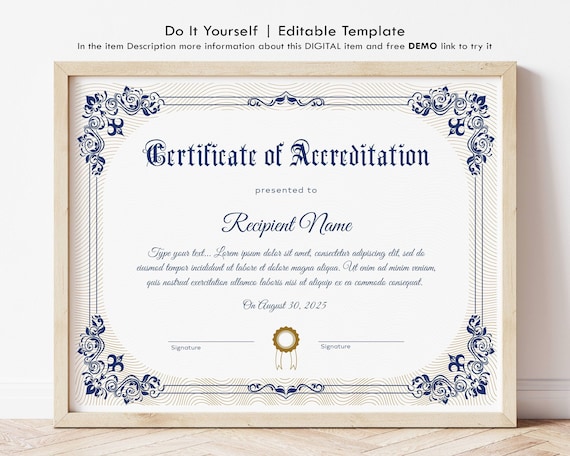This horizontally oriented, realistic image depicts a mock certificate of accreditation against a white wall and resting on a wooden floor. The certificate is displayed in a light-colored wooden frame, possibly resembling balsa wood or sandalwood. The main heading on the certificate reads "Certificate of Accreditation" in a dark blue, medieval gothic-style font. Below this title, it states, "presented to recipient name" in a larger font, followed by a placeholder Latin paragraph in an italicized font indicating where personalized information could be added. 

The certificate includes a sample date, "on August 30th, 2023," and beneath that, space for two signatures, each marked by the word "signature" below a line. Decorative elements adorn the document, including ornate, flowery symbols in all four corners and additional illustrations in the center and center bottom.

Above the frame, text in black reads, "do-it-yourself, editable template," suggesting the certificate can be customized. Below this, the item's description encourages users to explore more about this digital item with a free demo link provided. This advertisement highlights the editable nature of the certificate, implying its suitability for various personalized uses.